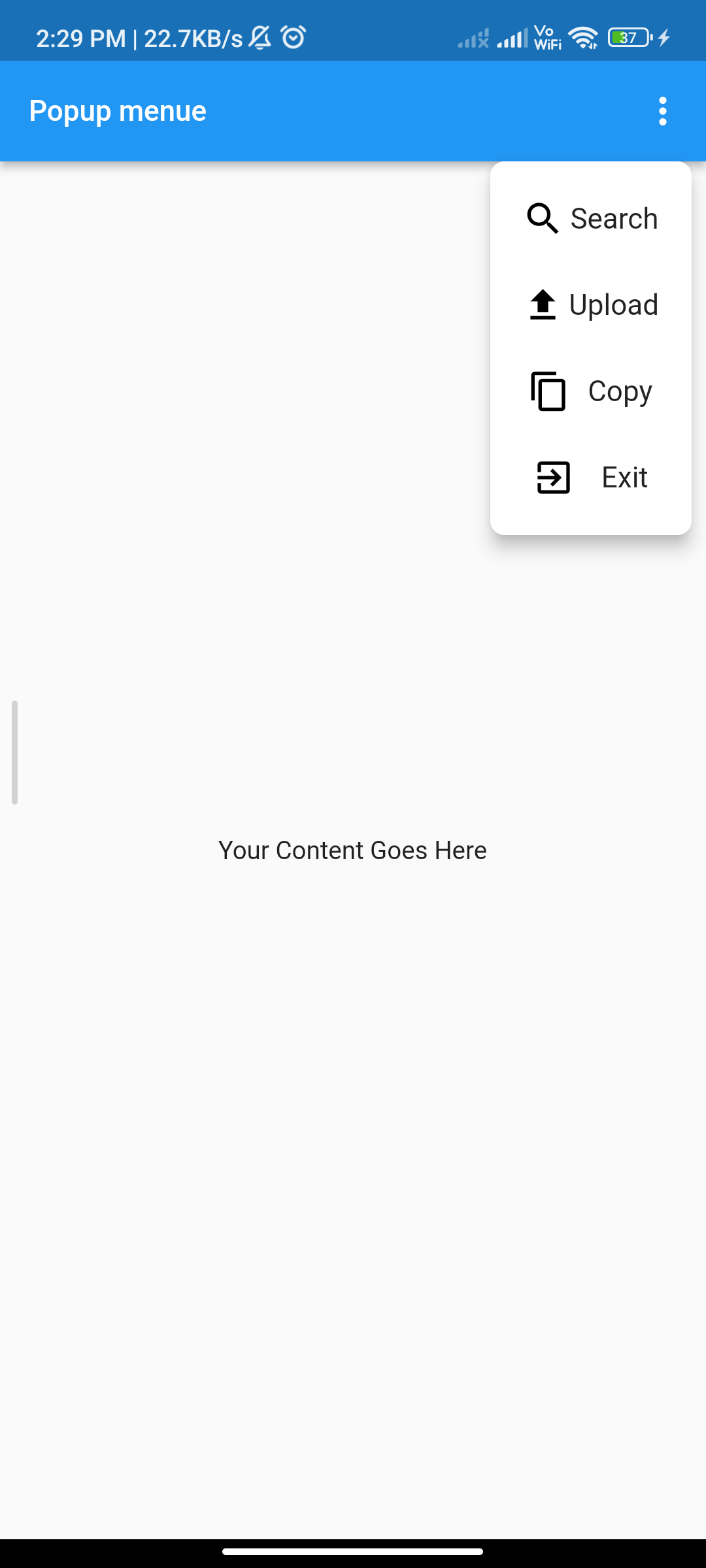This image, captured from a cell phone screen, provides a detailed view of a specific app's interface. At the very top, two horizontally aligned blue rectangles are visible. The upper rectangle is a darker shade of blue and slightly thinner, while the lower rectangle is a richer royal blue and a bit thicker. Displayed between these rectangles is the time, indicated as 2:29 p.m.

In the top left corner, several icons are present, though they are not specified. On the right, the icons include a battery indicator showing the battery level at 37%, with the percentage highlighted in green and accompanied by a lightning bolt symbol, signifying that the phone is charging.

Beneath these top sections, there's a lighter blue rectangle labeled "Pop-up Menu," and at its far right, three vertical white dots suggest additional options. Below this, a larger rectangle has expanded to reveal a menu with several functional icons: a magnifying glass labeled "Search," an upward-pointing arrow labeled "Upload," a pair of papers labeled "Copy," and a rightward-pointing arrow labeled "Exit."

Further down, centrally located within the image, is the text "Your content goes here," positioned in the area designated as the back of the phone.